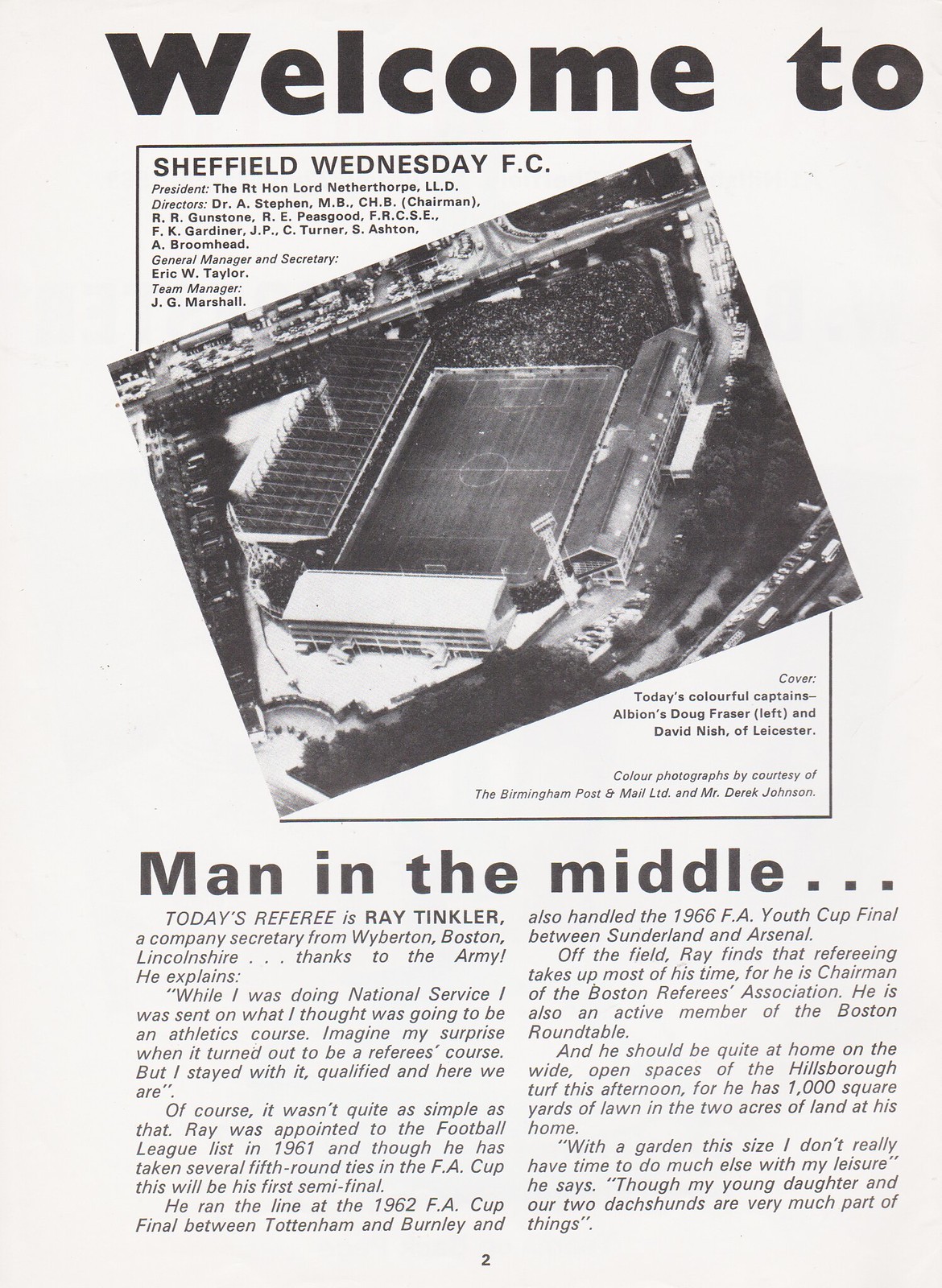The image appears to be a grayscale newspaper page or a game program related to soccer, specifically featuring content from a Sheffield Wednesday FC event. The top of the page prominently displays "Welcome to Sheffield Wednesday FC" in large, centered black text. Below this header, there is an aerial, slightly tilted, black-and-white photograph of a packed stadium, showcasing the stands, entrance, and the football pitch. 

The page continues to detail a section titled "Man in the Middle," which introduces today's referee, Ray Tinkler, a company secretary from Wibberton, Boston, Lincolnshire. The text recounts Tinkler's unexpected journey into refereeing during his National Service, where he mistakenly joined a refereeing course instead of an athletics course. Tinkler's refereeing career highlights include being appointed to the Football League list in 1961, officiating fifth-round FA Cup ties, and participating in significant matches like the 1962 FA Cup Final and the 1966 FA Youth Cup Final.

Off the field, Ray Tinkler devotes much of his time to his role as chairman of the Boston Referees Association and as an active member of the Boston Round Table. The feature adds a personal touch, describing his home life with his young daughter and two dachshunds, and noting his extensive gardening endeavors with 1,000 square yards of lawn and two acres of land. The page concludes with this being identified as page two of the program, emphasizing the professional and serious tone with black text against a white background. 

Notably, the page also credits the color photograph to the Birmingham Post and Mail Limited and Mr. Jack Johnson.